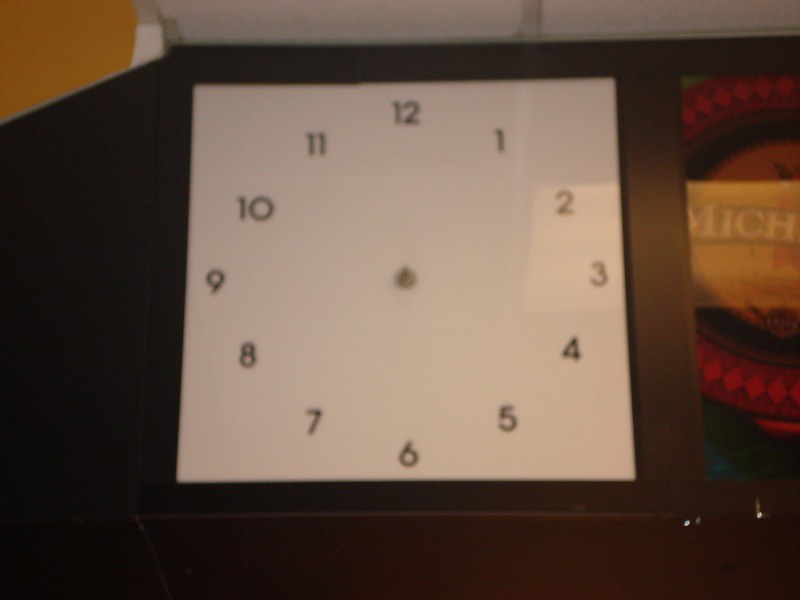This photograph depicts a somewhat blurry, incomplete clock face with a square, brown frame that appears to be made of wood or plastic. The clock face itself is white, displaying black or brown numbers from 1 to 12 arranged in a circular pattern around a small, central silver dot, but it lacks minute, second, or hour hands. The clock is resting on what seems to be a brown wooden surface. To the right of the clock is a partially visible object that might be a box, featuring yellow letters that seem to spell out "IMCH" or "MICH" on a yellowish-brown background. Additionally, there is a plate next to the clock decorated with orange or red triangles or diamonds.